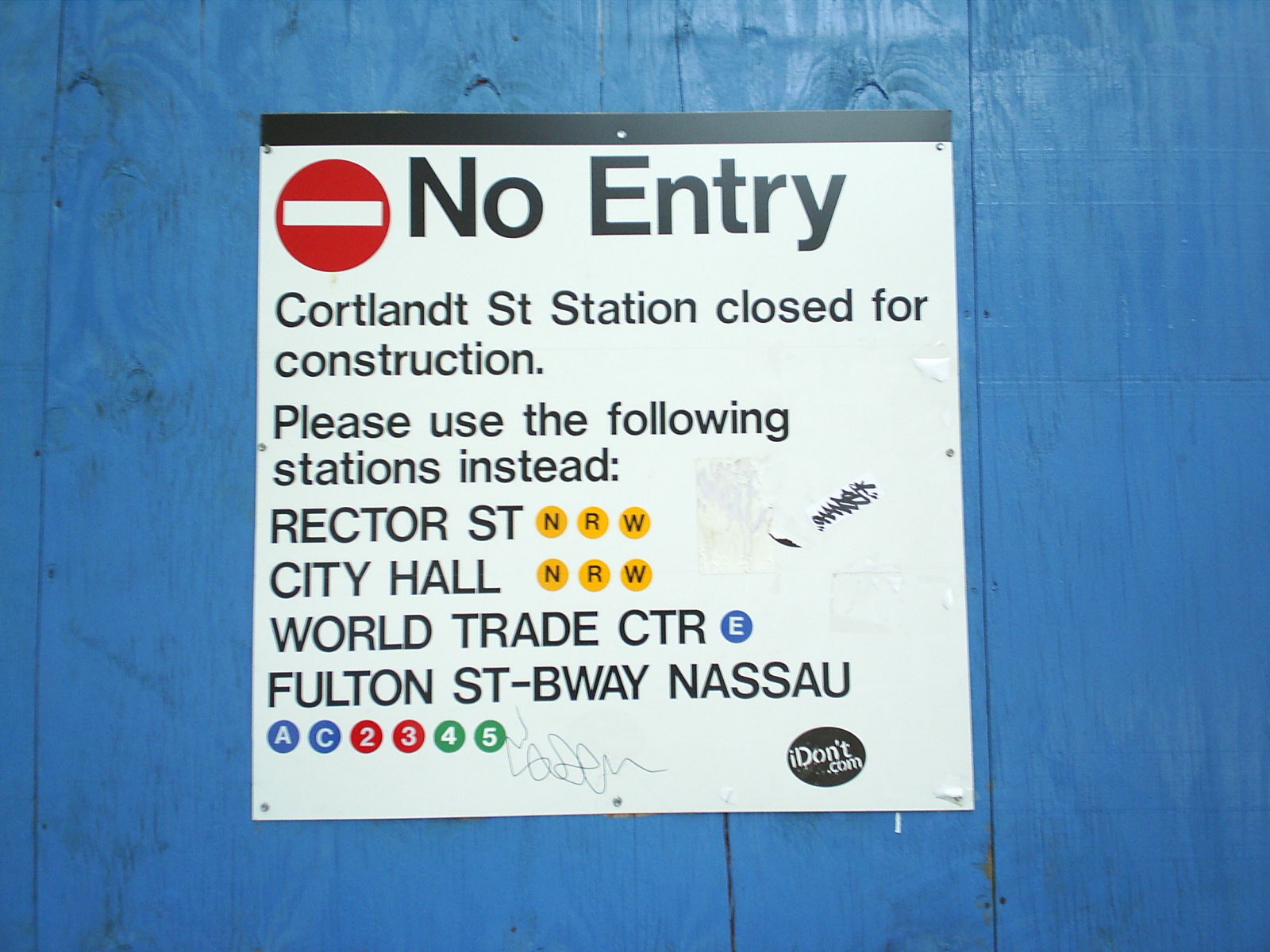The image depicts a large cautionary sign mounted on a high wooden fence made of light blue painted planks, resembling a sky-blue wall. This white sign, which appears to be either screwed or nailed into the blue paneling, is topped with a black rectangle and features a prominent red circle with a white dash, indicating "no entry." The sign reads: "No entry. Cortlandt St. Station closed for construction. Please use the following stations instead: Rector Street, City Hall (NRW in yellow circles), World Trade Center (E in a blue circle), Fulton St-Bway Nassau (C, 2, 3, 4, 5 in various colored circles)." The bottom right of the sign includes the text "idont.com," which appears to have a bit of graffiti or a scribbled signature beside it, suggesting some defacement.